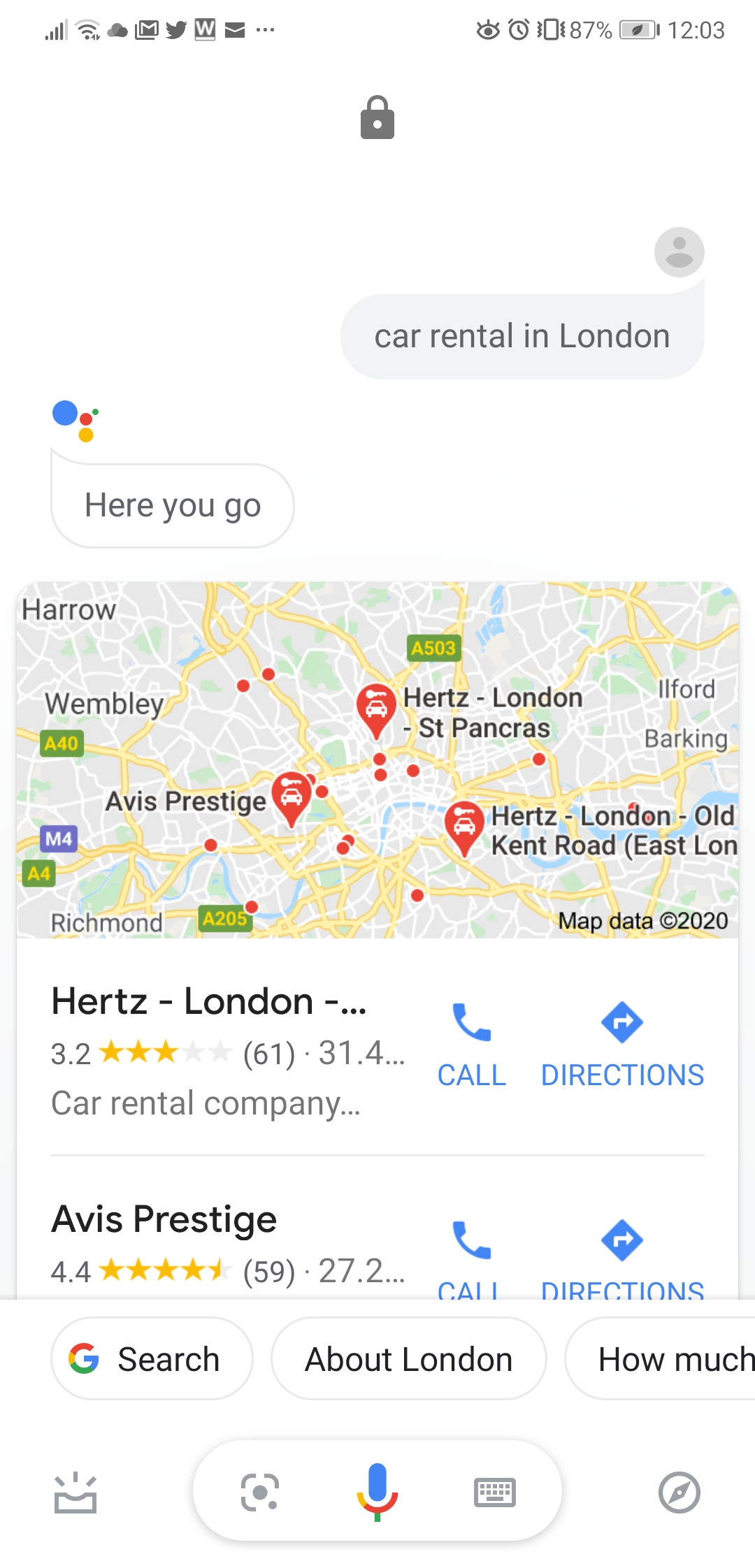This detailed screenshot, likely from an Android device as suggested by the notification icons in the top-left corner and general app layout, captures a search query made via Google Assistant for "Carbuncle in London." In response, Google Assistant presents several relevant results, prominently featuring car rental locations in London.

The first visible result is "Hertz London," pinpointed on a map along with other options. The primary listings detailed on the screenshot include:
1. **Hertz London, St. Pancras**: This entry boasts a 3.2-star rating based on 61 Google reviews and seems to be approximately 31.4 kilometers away. There's an option to either call or get directions, both highlighted in blue buttons.
2. **Avis Prestige**: This alternative offers a higher 4.4-star rating from 59 reviews, with an estimated distance of around 27.2 miles. Similar to the previous entry, it also features blue call and direction buttons.

Additionally, a partially visible search bar at the bottom of the screen includes an incomplete query about London, alongside a series of interactive buttons. These encompass a microphone icon in Google colors for voice searches, a camera search option, a keyboard input option, and a couple of other utility buttons bracketing the central controls.